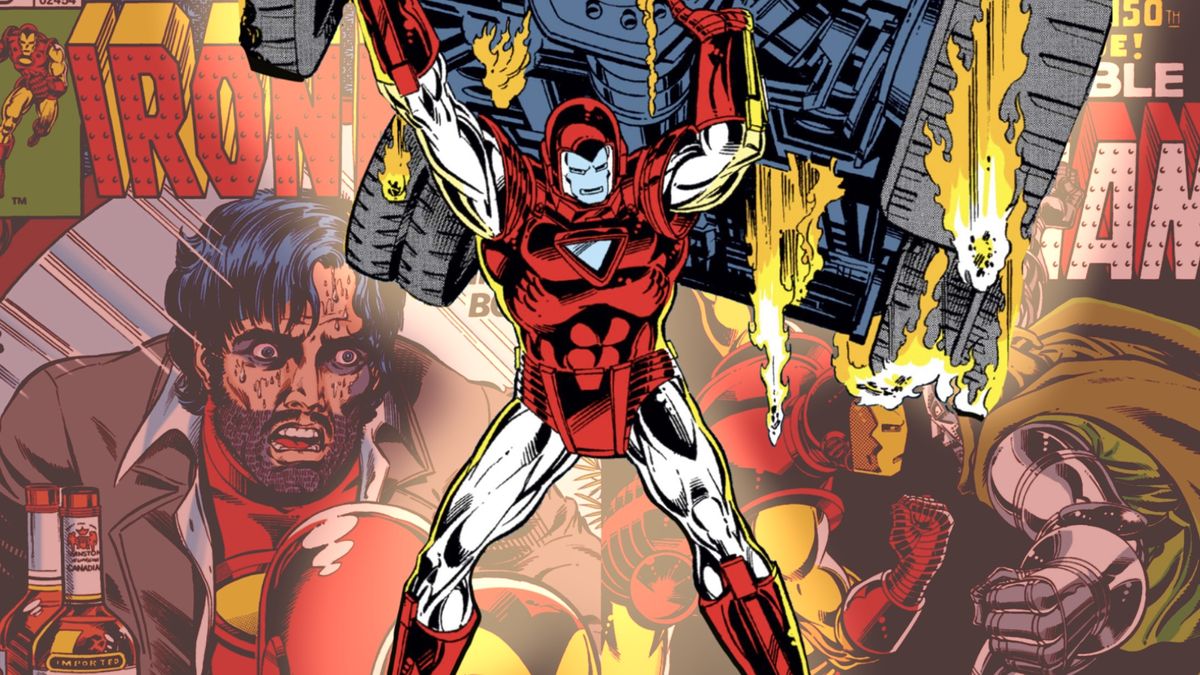This image is an intricate comic book cover from the Iron Man series, featuring the titular hero. At the center, Iron Man, clad in a striking red and yellow metal suit with white accents on the arms and face mask, is depicted with remarkable muscle definition. He is dramatically lifting and throwing a heavily detailed black military vehicle or tank, which is engulfed in vivid yellow flames, emphasizing the intense action sequence. On the bottom right, Iron Man is engaged in a fierce face-off with Doctor Doom, identifiable by his metallic suit and cape. On the bottom left, there’s a detailed illustration of Tony Stark, discernible with black, sweat-soaked hair, wide eyes encircled by dark rings, and a brown jacket that partially reveals the Iron Man suit underneath. The text "Iron Man" is prominently displayed in bold red letters, with parts extending over to the right in white, creating a dynamic and visually compelling design that embodies the high-energy and heroic essence of Iron Man.